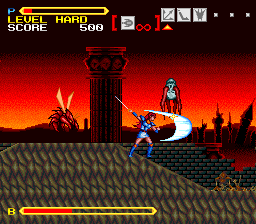This screenshot captures an intense moment from a video game. In the top-left corner, a yellow power meter and a red progress bar—barely filled—are visible. The words "Level: Hard" appear in yellow text just above a "Score: 500" display in white. At the center of the screen, a blue-armored character brandishes a silver sword, seemingly engaged in a duel with a nearby red ghost or monster. The backdrop features a striking combination of a red sunset merging into a dark, blackened sky above, setting a dramatic and ominous stage for the encounter.